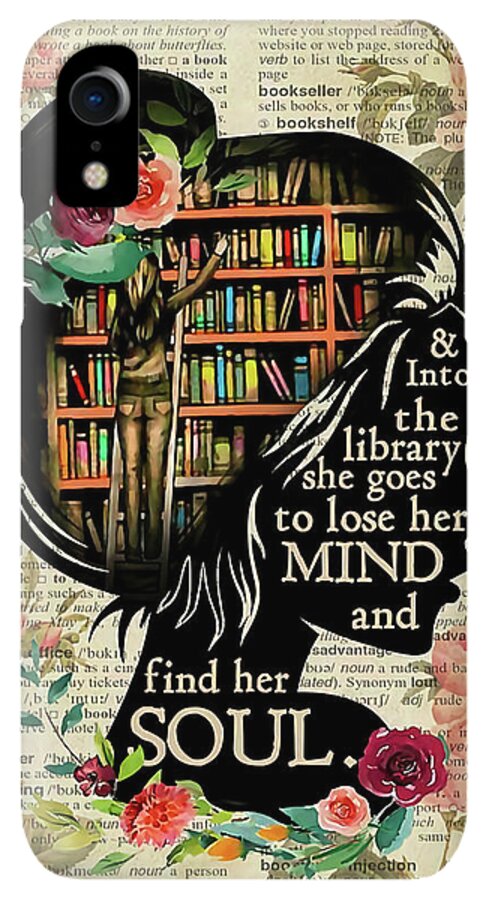The image appears to be an advertisement for a library, promoting a social service where one can learn and immerse in literary adventures. The background features a partial page from a dictionary, with bolded words, pronunciation symbols, and definitions. Overlaying this background is a detailed illustration of a woman with her face in silhouette, facing right, and adorned with a floral barrette in her bun. The silhouette contains a scene where the woman is on a ladder, reaching for a book on a six-level, old-fashioned bookshelf filled with multi-colored books. There are floral illustrations beneath her chest and around her hair, adding a decorative touch with red, pink, and orange flowers forming an arch. Text in white letters on a black background within the silhouette reads, “Into the library she goes to lose her mind and find her soul.” A smartphone with a camera icon is depicted in the top left, suggesting that the image might be interactive or can be looked up with a phone. The overall color scheme includes pink, peach, green, blue, light yellow, black, and off-white, creating a vibrant and inviting atmosphere.